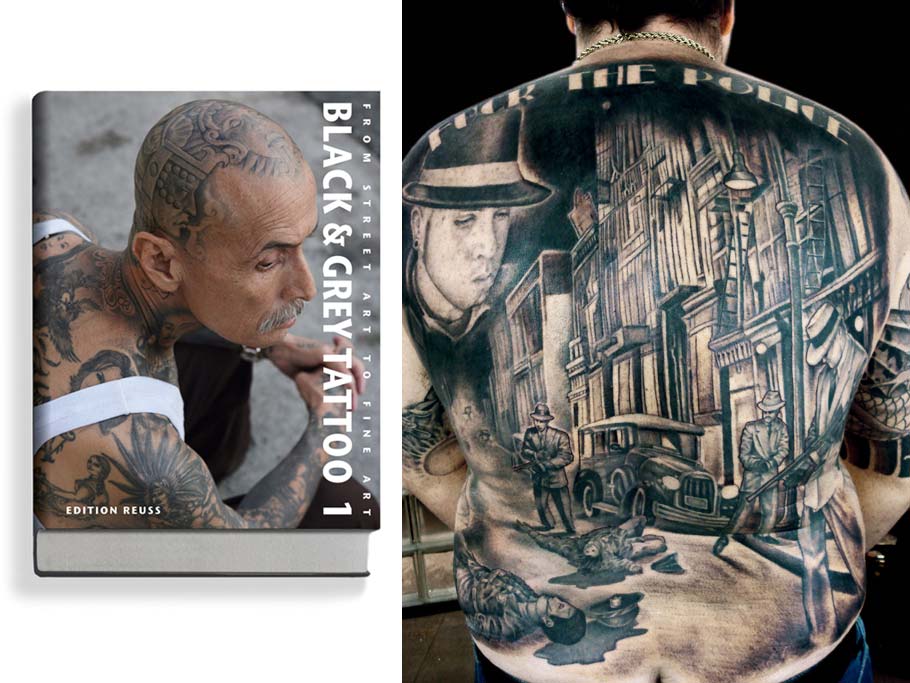This split image features on the left an angled photograph of a book cover in color, titled "From Street Art to Fine Art: Black and Gray Tattoo 1." The book showcases a heavily tattooed older gentleman wearing a white sleeveless shirt, revealing an intricate array of black and gray tattoos covering his bald head, neck, right arm, back, and part of his left shoulder. He is seated, donning black pants, and gazing slightly to the right. Written in white along the bottom of the cover is "Edition Roofs."

The right image spotlights an extensive back tattoo on a man, featuring a dramatic scene reminiscent of the 1920s-1940s era. Crowning the tattoo design is the phrase "F the police." The artwork includes detailed depictions of men in suits and hats wielding Tommy guns, and lifeless bodies lying in pools of blood, signaling a violent confrontation. A vintage car with its lights on and a white top is also present in the background. On the man's top left shoulder blade is a realistic portrait of a man with long sideburns, sporting a hat with a ribbon, and an earring. The bottom of the image reveals the man wearing jeans slightly lowered, exposing the top of his buttocks.